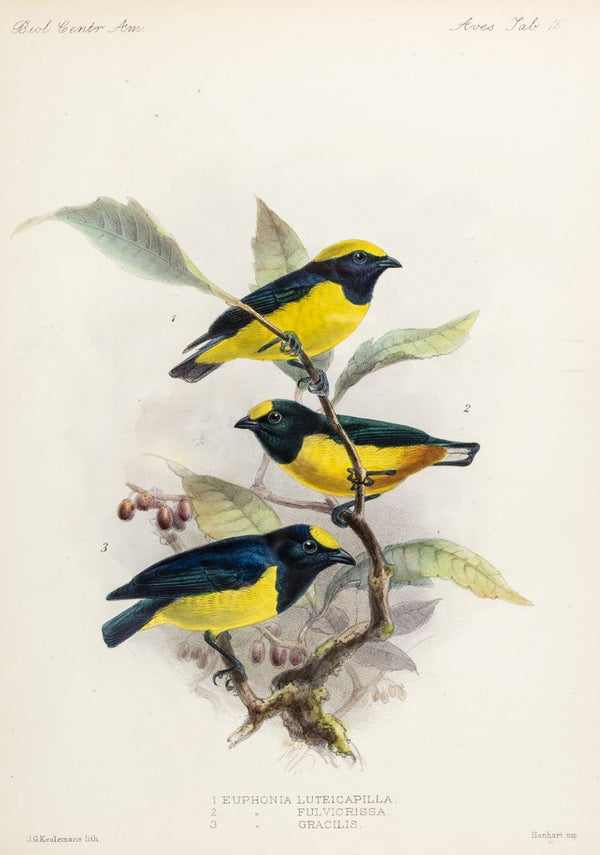The illustration depicts three small birds perched on a tree branch with several leaves and oval, purple fruits. The background is a white or off-white color. The birds are primarily black and yellow, with black feathers on their wings, tails, and most of their heads. They have black beaks that extend towards their black feathers, with yellow patches around their eyes and on the undersides of their bodies. The birds are positioned side-by-side, with the two outer birds facing right and the middle bird facing left. Below the illustration, text labels identify the birds, though the exact names appear to be in Latin and include species such as "euphonia luteicapilla," "euphonia fulviris chica," and "euphonia graschilis." The predominant colors in the image are black, yellow, shades of dark and light green, and brown.